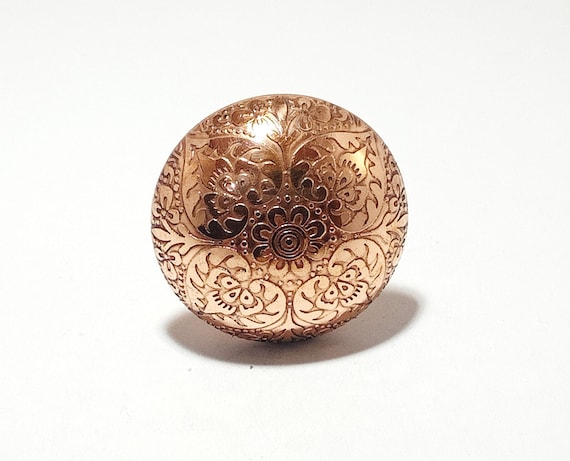The photograph captures a medium-sized, intricately carved golden ball set against a plain white background. The ball's metallic gold surface gleams as if recently polished, casting a subtle shadow underneath. Its elaborate design features an array of floral patterns, hearts, loops, and other ornamental motifs, all raised and textured, giving it a distinctly embossed or engraved appearance. While the object is circular and could potentially be a bead or button, it's primarily depicted as a beautifully detailed golden ball, showcasing its ornate craftsmanship and singular, metallic gold coloration.